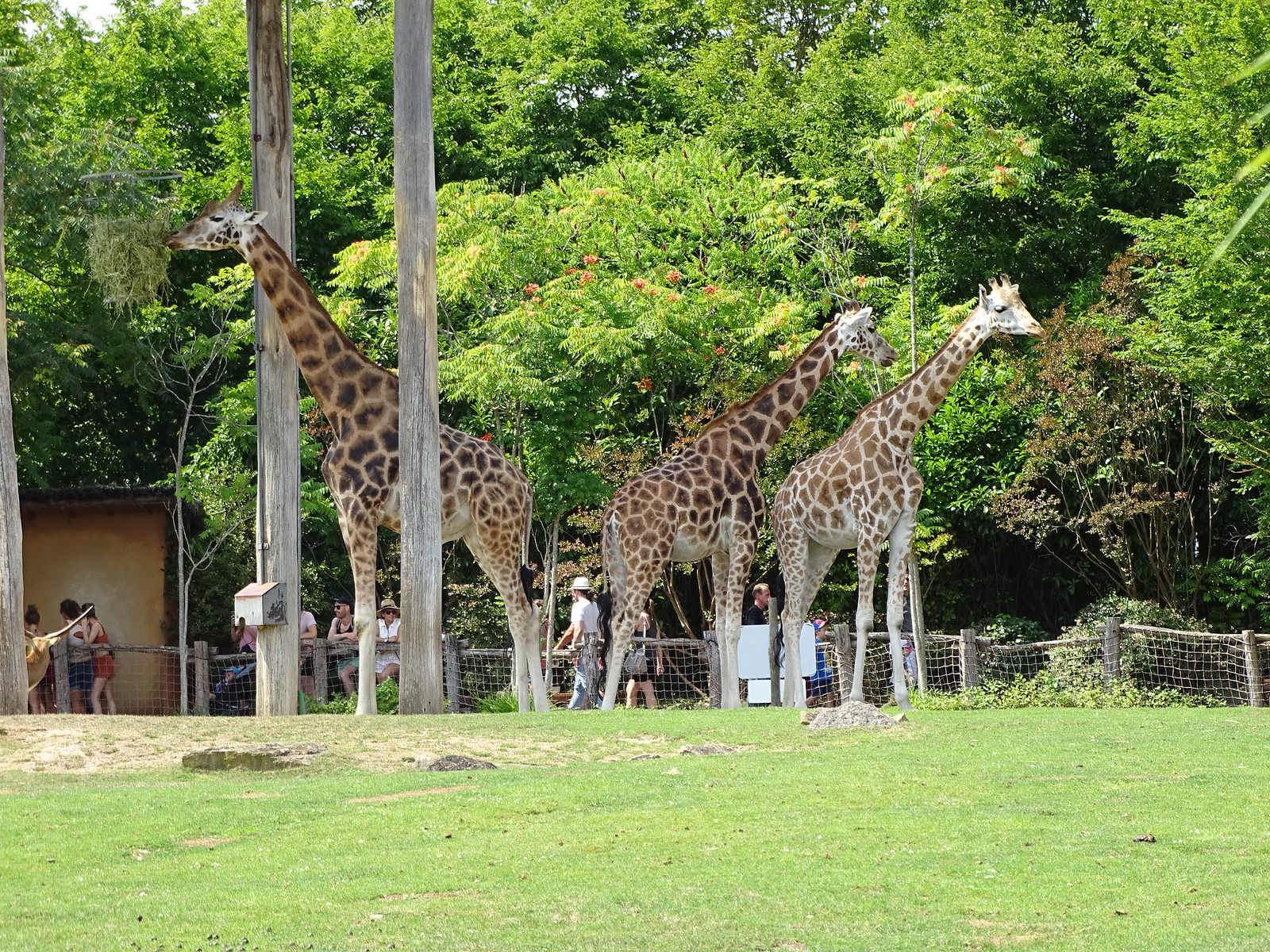In this color photograph taken at what appears to be a zoo or wildlife park, three giraffes stand in a grassy enclosure. The giraffe on the left is positioned between two tall wooden poles, one of which has a box attached to its lower side. This giraffe faces left, looking towards the left side of the image. The other two giraffes face right, observing their surroundings. Beyond the low wooden fence of their enclosure, zoo visitors can be seen walking or leaning against the fence, watching the giraffes. The enclosure is backed by tall, leafy green trees, one of which bears red flowers. To the far left of the image, a small shaded structure shelters three people engaging in conversation. Overhead, the sky is a clear blue, visible through the gaps in the trees.